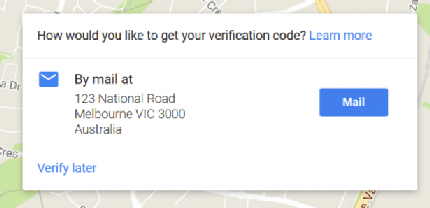The image is a rectangular screenshot, approximately 30:70 in height-width ratio, capturing a segment of a digital map, likely from Google Maps, based on the recognizable color scheme. The background map features predominantly gray areas with several green patches indicating parks. A yellow curving highway stretches upwards, accompanied by a few delineated white streets.

Overlaid on this map is a horizontal white box containing text and graphical elements. At the top, in black text, it reads, "How would you like to get your verification code?" Next to this, in blue text, is a "Learn more" link. Below, a thin gray line spans the width of the box, providing a visual divider.

Underneath the line, it displays in black text, "By mail at 123 National Road, Melbourne, VIC 3000, Australia," with a small blue envelope icon to the left. At the bottom left of the box, "Verify later" is written in blue text. On the right-hand side, there is a rectangular blue button with "Mail" inscribed in white text, indicating an option to choose for receiving the verification code.